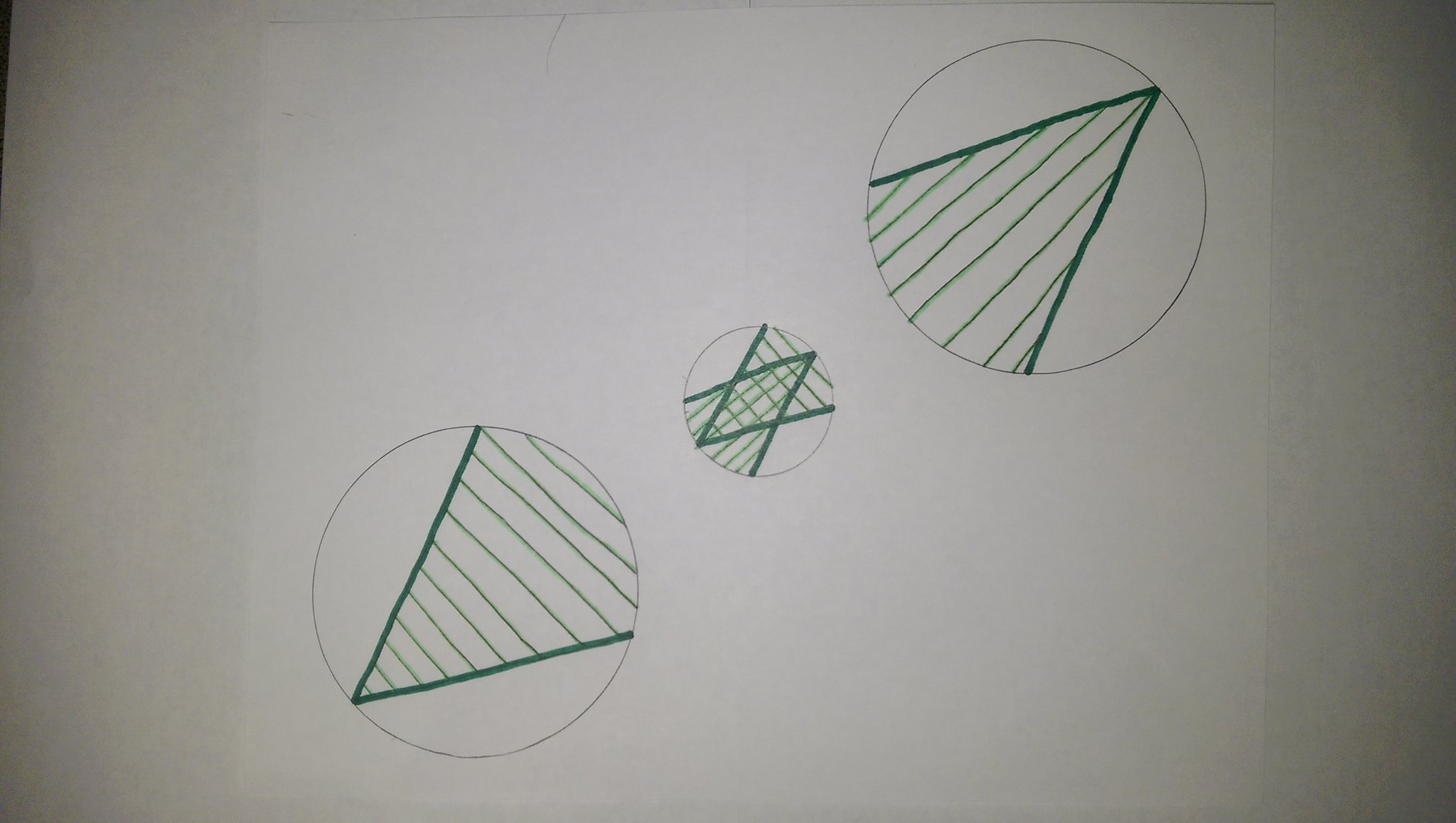This photograph captures a meticulously detailed sketch on a piece of white paper, which appears gray due to poor lighting. The gradient shading of the image causes the left and right edges to be darker gray, and the four corners to nearly fade into blackness.

The focal point of the sketch features two large circles, one positioned toward the bottom left and the other toward the top right, with a smaller circle nestled in the center of the composition. 

In the bottom left circle, a bold V shape points towards the bottom left corner. This V is intricately filled with horizontal lines that run parallel and uniformly across the shape, halting at the curved border of the circle.

Contrastingly, in the top right circle, another V shape points towards the top right corner. Within this V, vertical lines span from one edge to the other, maintaining a parallel alignment with each other.

Centrally, within the smallest circle, the artist has cleverly combined the two V shapes. In this arrangement, the V shapes are inverted and superimposed to create a striking diamond pattern adorned with a grid-like structure formed by intersecting horizontal and vertical lines. The intricate detail and symmetry of this central design draw attention to the precise craftsmanship of the sketch.